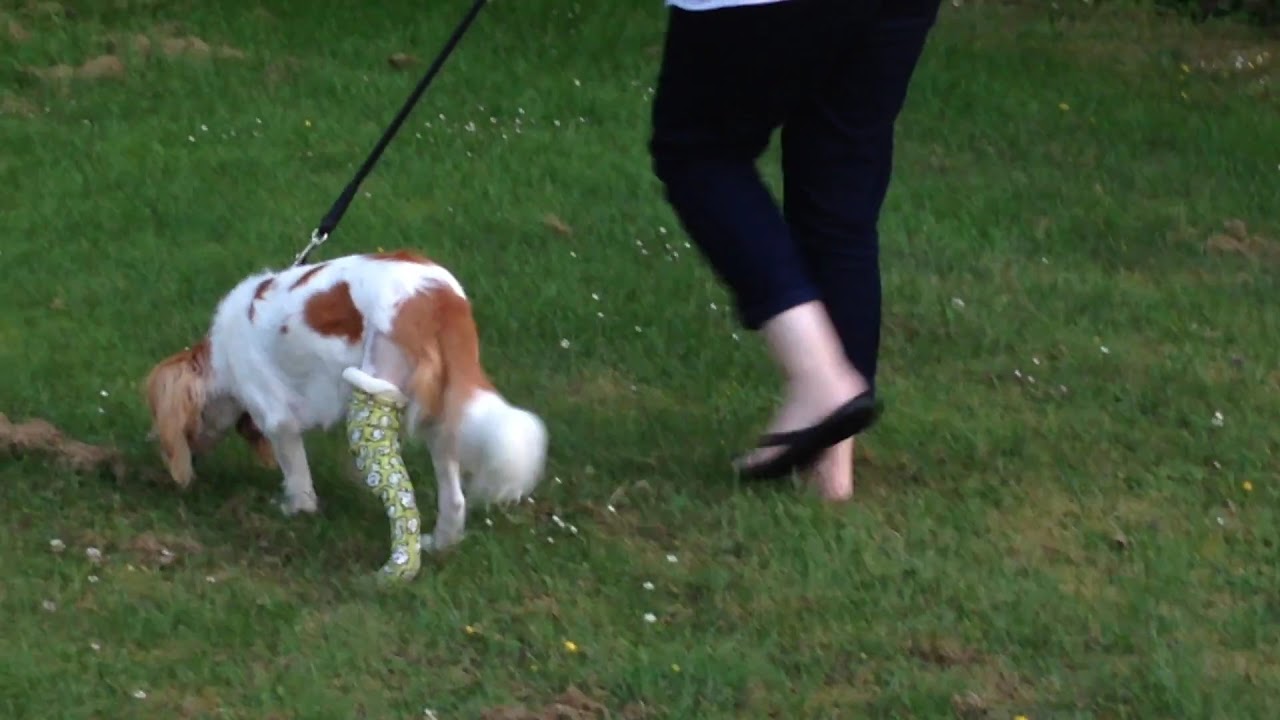The image captures an outdoor scene, likely taken during the daytime, featuring a grassy field interspersed with clover and patches of brown grass. In the center, the bottom half of a woman is visible, clad in dark blue, cropped trousers and black flip-flops, without socks. She appears to be taking a step with her left foot. A black leash extends from her left hand at an angle, connecting to a reddish-brown and white spotted spaniel-type dog positioned slightly to her left. The dog faces away from the camera, its head bent down as though sniffing or eating something on the ground. Notably, the dog's back left leg is encased in a green and white cast, with a shaved area of fur visible just above it. The dog has brown floppy ears and a tail tipped with a bushy white end.